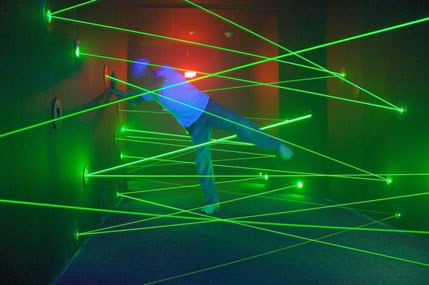A computer-generated image shows a man in a dark room intricately navigating a maze of green laser beams crisscrossing from circular portholes on red and green walls, with a blue floor. The green beams primarily emerge from irregular patterns of circular openings and span from wall to wall, cutting the room into an intense, high-stakes web of light. The man, dressed in a white t-shirt, jeans, and a white English derby hat, skillfully balances on one leg while bracing himself sideways against one wall, expertly dodging the lasers. His left leg is elevated at an angle, demonstrating a careful maneuver to avoid breaking the waist-high beams that shoot in various directions—upward, downward, backward, and forward. The room's background features additional red lighting, enhancing the vivid contrast of the scene and highlighting the perilous, game-like challenge he faces.